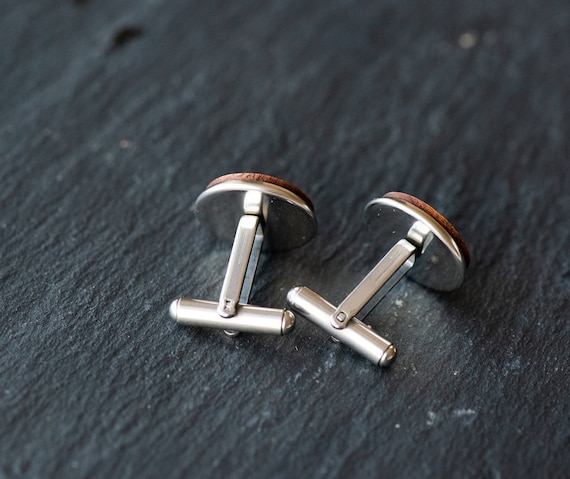The image features two silver, T-shaped objects resembling cufflinks, positioned upright on a black, textured surface with ridges. Each object has a round, chestnut-colored end, which could be wooden, providing a distinct contrast to their metallic bodies. The cufflinks are nearly touching, aligning side-by-side, giving the impression that they can rotate on their axes. Their setting and the focus on the detailed elements suggest a close-up, squared composition, typically used for showcasing small items like tools or accessories.